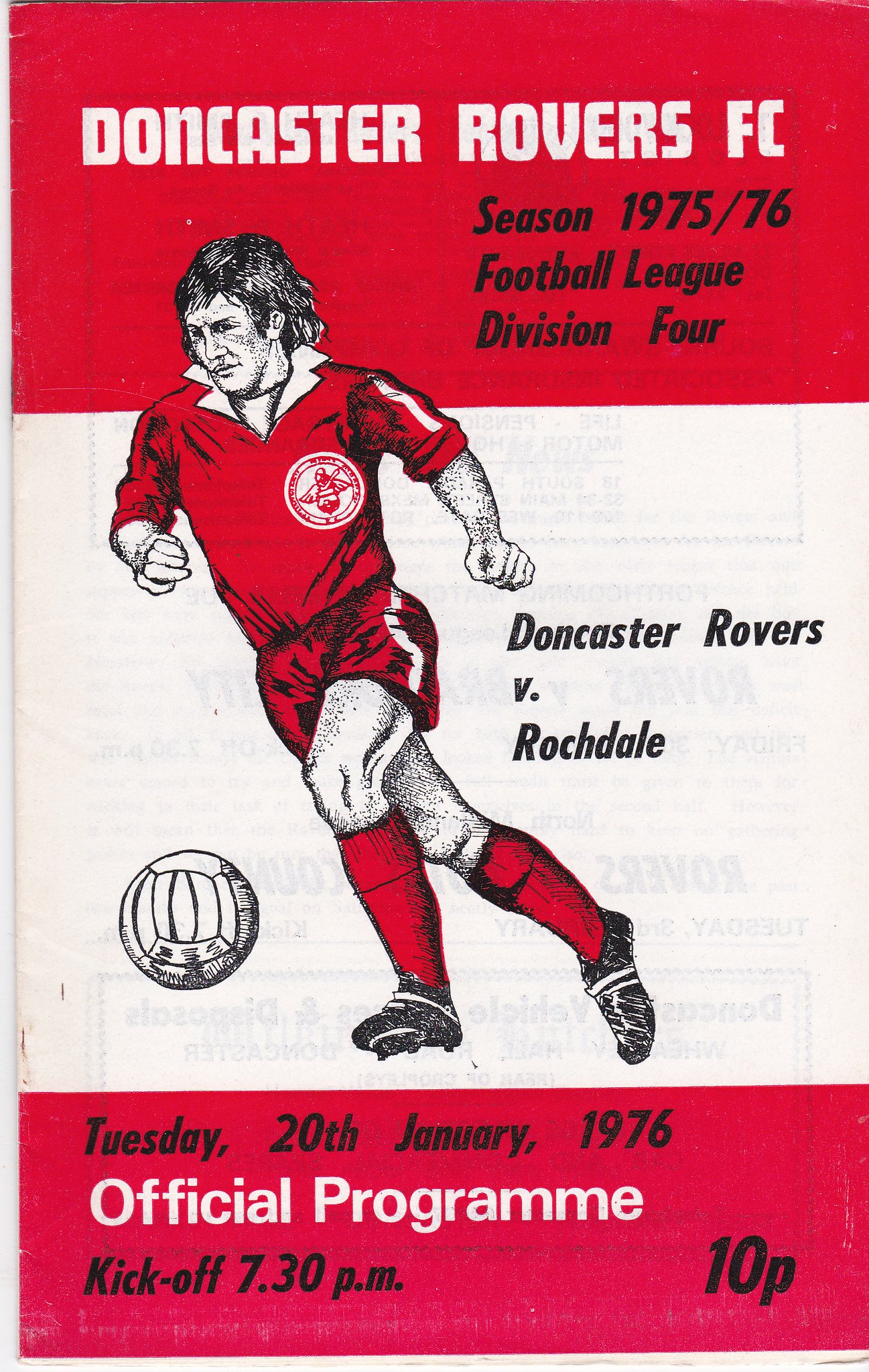This vintage soccer league program, dated for the 1975-76 season, features a predominantly red and white color scheme with elements of black and gray. The cover prominently displays hand-drawn artwork of a soccer player in a red uniform with cleats and red stockings, energetically kicking a soccer ball positioned on the left side. The player, depicted with a concentrated expression, is central to the design but slightly offset to the left. Surrounding this illustration, various texts identify the program's details in a mix of white and black lettering.

At the top in white print, it reads "Doncaster Rovers F.C." Beneath this, in a black right-slanted script, "Season 1975-76, Football League, Division IV" is indicated. The match specifics, "Doncaster Rovers vs. Rochdale," appear to the right of the player. Lower down, the red section contains the match date and time: "Tuesday, 20th January 1976," with "kickoff 7:30 p.m." scripted in black. At the very bottom right, the price is noted as "10 pence" in smaller white print. This program epitomizes an era preceding digital design, exuding a nostalgic, handcrafted charm.